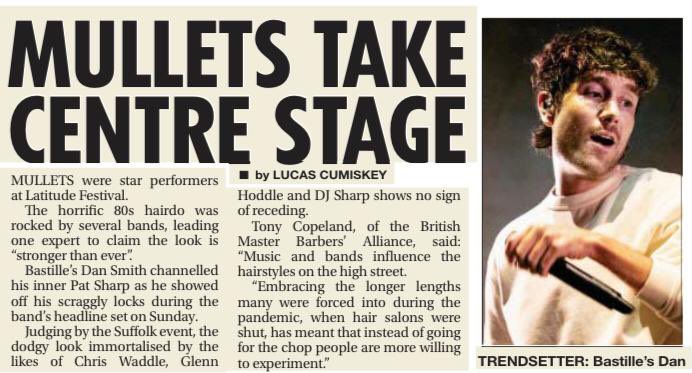This is a detailed newspaper clipping headlined, "Mullets Take Center Stage" by Lucas Kaminsky, written in prominent black lettering on a white background. The article discusses the revival of the notorious 1980s haircut, particularly highlighted at the Latitude Festival where several bands sported the mullet. To the right of the article is a color photo spanning its length, showing a young man named Dan Smith of the band Bastille. Dan, described as a trendsetter, is captured in the image wearing a white sweatshirt and holding a microphone while looking to his right, showing off his short mullet. The article cites expert Tony Copeland of the British Master Barber's Alliance, who notes that music and bands significantly influence street fashion. He explains that the pandemic's lockdowns led to people embracing longer hairstyles, making them more open to experimenting instead of opting for a short cut. This resurgence of the mullet, likened to styles worn by Pat Sharp, Chris Waddle, and Glenn Hoddle, suggests that the once-derided look is now stronger than ever.